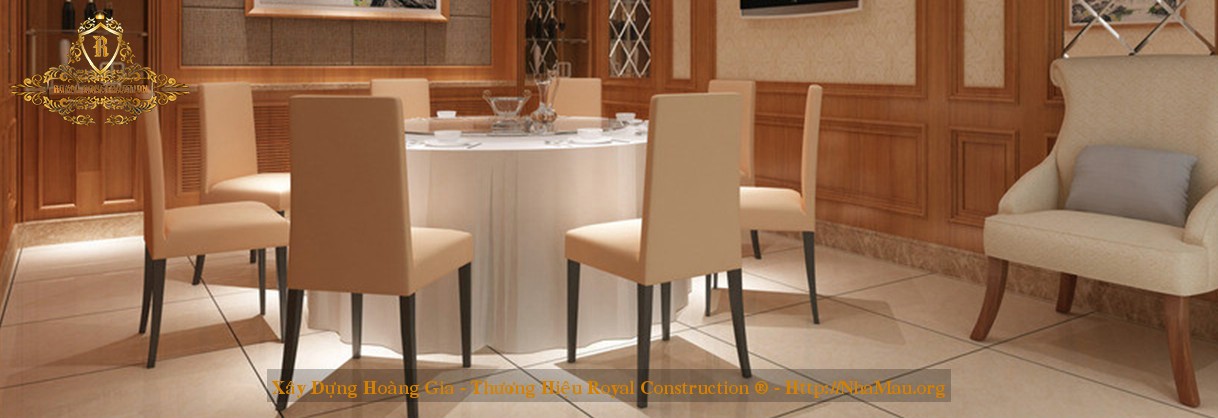This landscape photograph captures the elegant interior of a lavish setting, possibly within an upmarket hotel or restaurant, adorned with sophisticated furnishings. At the center, a round table draped with a pristine white tablecloth reaches down to the floor, surrounded by eight equidistantly placed, high-backed peach chairs with brown wooden legs. The table is meticulously set with glassware, cutlery, plates, and what appears to be either tiny soup bowls or teacups.

The floor is composed of large beige or peach-colored tiles, adding a touch of opulence to the room. To the left of the table, there's a large white armchair with four splayed wooden legs, accented by a gray pillow, enhancing the room's comfortable yet luxurious vibe. The surrounding walls feature rich wooden paneling topped with tan wallpaper, complemented by the presence of barely-visible framed pictures at the top of the image. 

Notable details include a refined logo in the top left corner featuring a capital "R" within a shield-like design adorned with frilly golds and green leaves, indicative of an affiliation with Kedong Huangjia Royal Construction, whose website and emblem watermark span the bottom of the image. This setting, with its combination of elegant design elements, suggests it is either an advertisement for high-end interior furnishings or a promotional image for a company specializing in luxurious hotel or restaurant construction and decoration services.